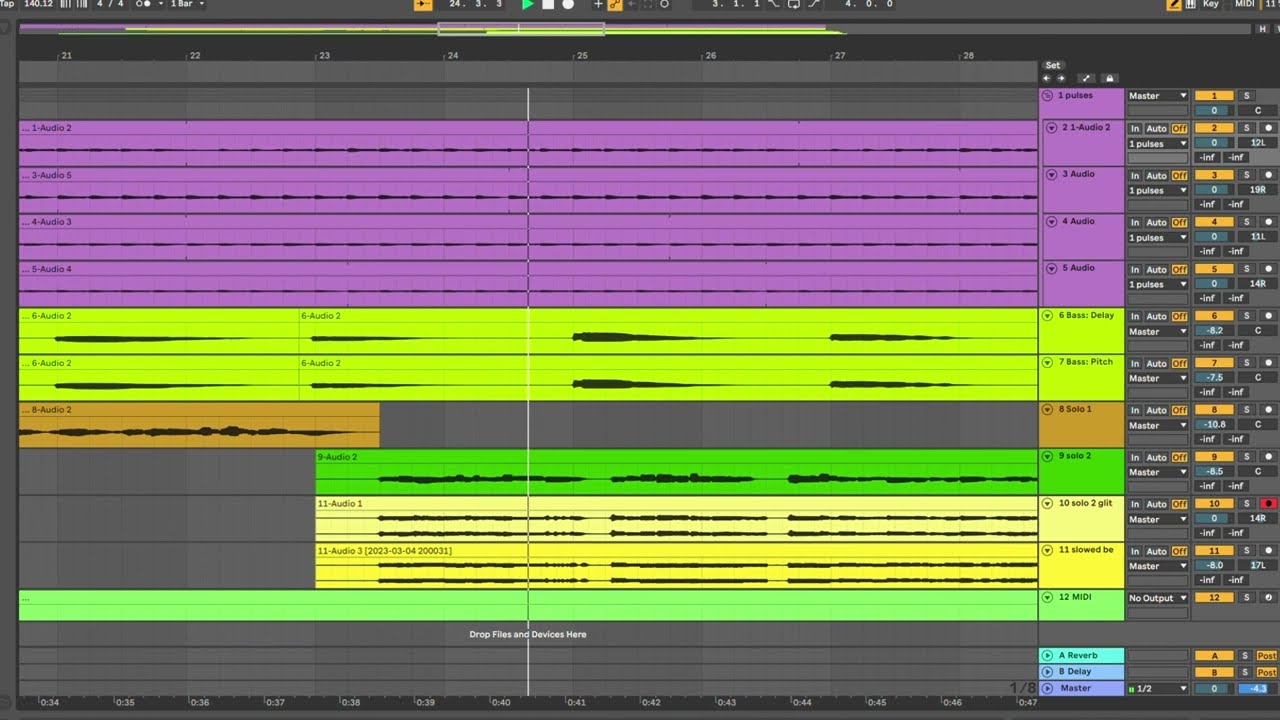The image is a detailed screenshot of a music production software interface on a desktop computer. The screen displays an electronic, computerized soundboard featuring multiple audio waveforms and levels, each identified by distinct colors. The background is dark, with the main colors being gray, green, and lavender. There are several rows of waveforms, starting with four lavender-colored layers at the top, followed by two mint green layers. Beneath these, there is a gold-colored waveform, which transitions to a standard green layer. Below this, there is a tan waveform followed by a yellow waveform, and finally, a sage green layer at the bottom.

The interface includes a bar running vertically from top to bottom, indicating the playback position and showing the audio levels spiking and dipping in response to the recorded material. At the top of the screen, menu icons for various functions are visible. Off to the right, there are detailed settings, possibly corresponding to twelve different audio tracks, as indicated by small lettering. Though the name of the program is not visible, the interface suggests a complex soundboard program designed for detailed audio editing and production.